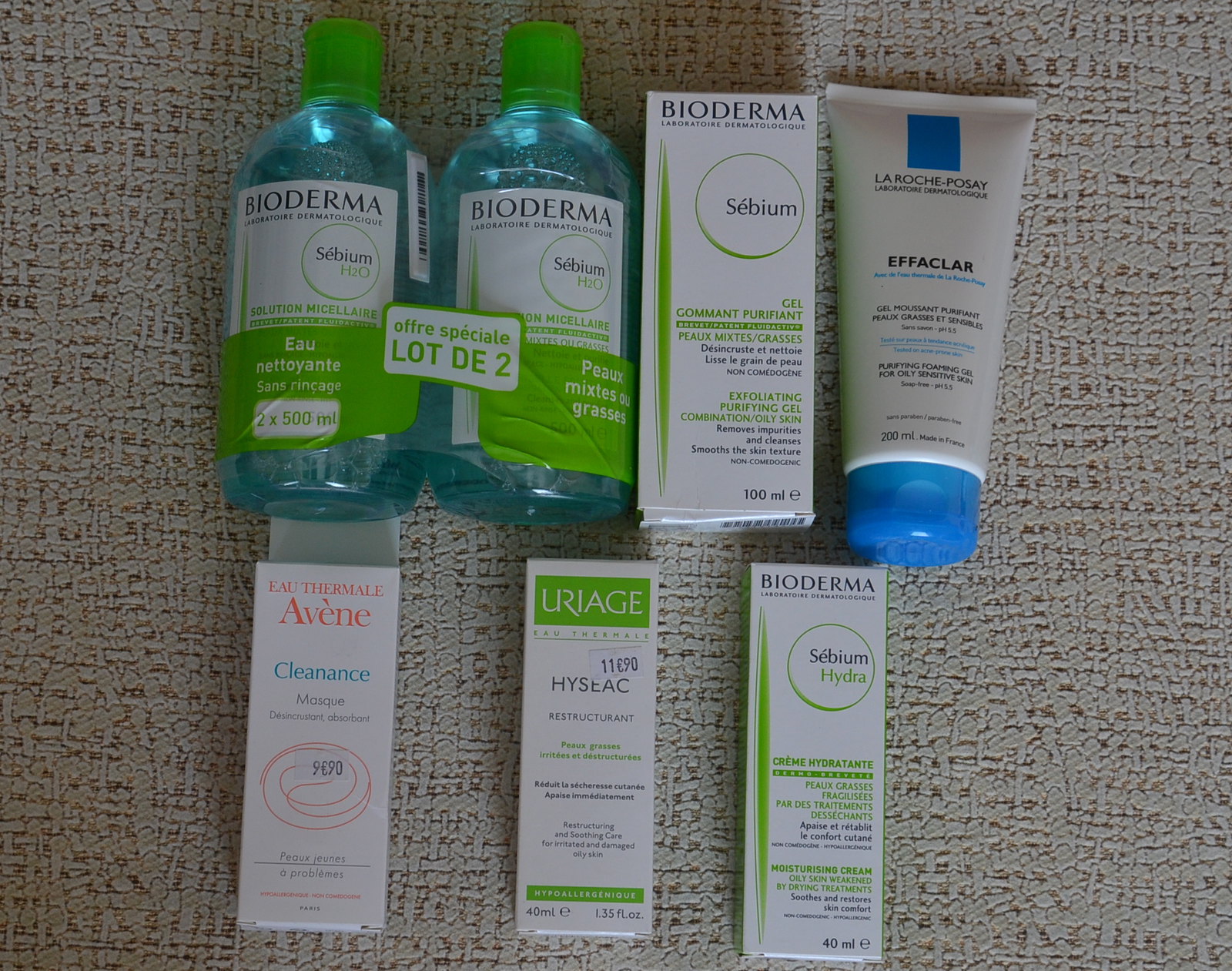Displayed on a textured fabric surface, which appears to be a tablecloth, is an assortment of skincare products. The eye-catching pattern of the tablecloth suggests a woven design, with non-symmetrical grooves that lend it a distinctive tactile quality.

At the top of the arrangement, two clear bottles with vibrant, bluish-turquoise liquid can be seen lying horizontally. Each bottle is capped with a green lid and labeled in French, featuring black and green text announcing the renowned brand Bioderma.

Next to these bottles is a vertical rectangular box, also from Bioderma, labelled with the sub-brand "Sebium," though the finer details of the text are difficult to discern.

Adjacent to the Bioderma items, there is a tube of Effaclar by La Roche-Posay, hinting at its skincare purpose, though the specific content remains unspecified.

On the bottom row, several boxed items complete the spread. The first box belongs to Avene and is marked with "Cleanance," suggesting it is part of their skincare line. Following it is a box from Uriage, labelled "Hyséac," again indicating skincare purposes. Lastly, another box from Bioderma features "Sebium," with "Hydra" noted on the label.

This collection of high-end skincare products seems poised for careful examination or use, each promising different benefits to the discerning user.